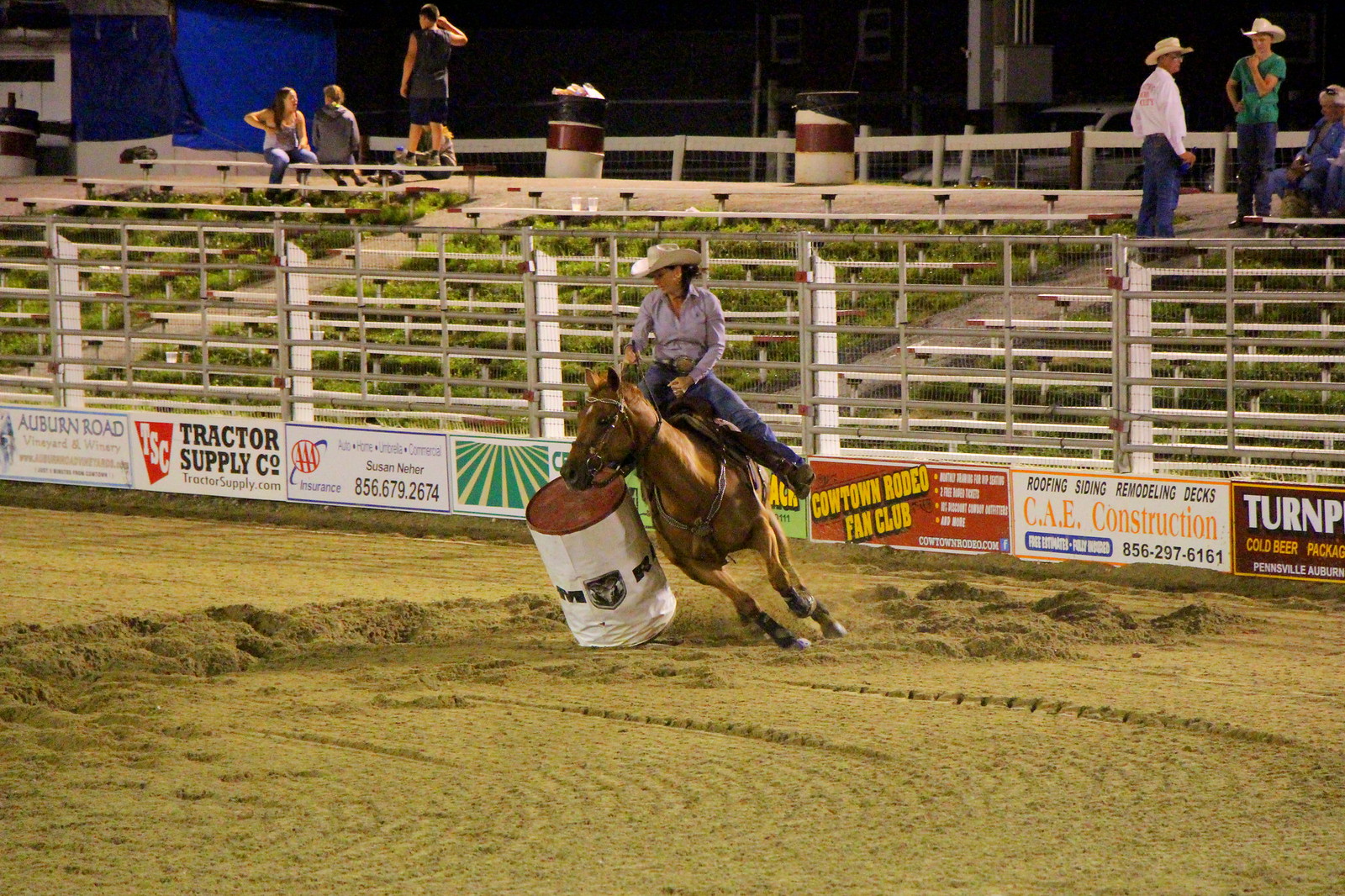This nighttime rodeo photograph captures a dynamic scene inside a well-lit, small stadium with about six or seven rows of sparse bleacher seats. At the center of the dusty, olive-toned field, a young woman dressed in jeans, a long-sleeve shirt, and a cowboy hat skillfully rides a brown horse around a white barrel emblazoned with black lettering. The background features several advertisements, including a prominent one for Dodge truck manufacturers, as well as sponsors like Tractor Supply Company and the Caltown Rodeo Fan Club.

Despite the sparse attendance, the diverse crowd includes a few individuals in cowboy hats and some spectators in summer outfits, suggesting a warm night in Texas. At the top of the bleachers, there are visible trash cans and a group of children on the left side. The horse and rider are captured in mid-motion, highlighting the energy and action of the rodeo event.